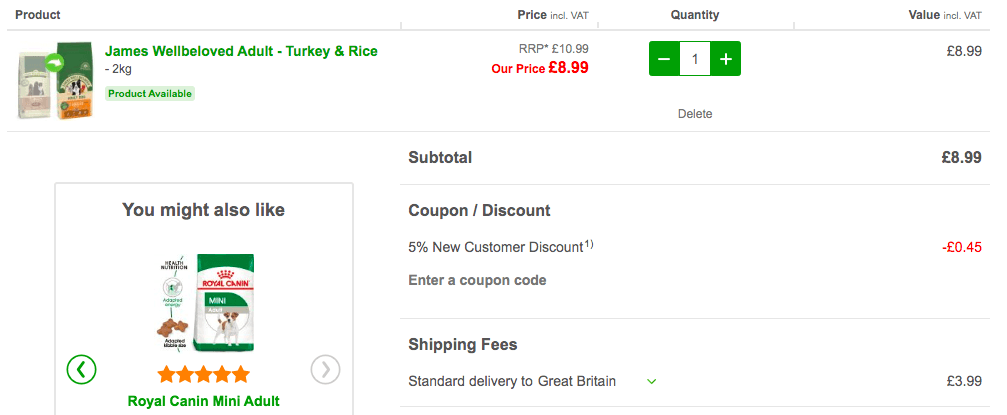**Detailed Product Page Description:**
------------------------------------------

The webpage resembles an online retail platform specializing in dog food. It features a clear, white background with predominantly black text, offering a clean and visually accessible layout.

**Header Section:**

- **Title:** At the top of the page, the word "Product" is prominently displayed.
- **Image Slider:** Below the title, there are images of dog food bags, predominantly green and yellow-orange in color, showcasing the products available.

**Main Product Information:**

- **Brand and Product Name:** To the right of the images, the text reads, "James Well-Beloved Adult Turkey and Rice."
- **Weight and Availability:** Below this, it mentions "2 kilograms product available," highlighted in green.
- **Price:** Next to the availability, the price is clearly labeled with a pound symbol, "£8.99."

**Quantity Selection:**

- **Adjustable Quantity:** The webpage features a user-friendly quantity selector. The default amount is "1," with "-" and "+" buttons on either side allowing the user to decrease or increase the quantity as required.

**Subtotal and Value:**

- **Total Value:** Adjacent to the quantity selector, there is a "Value" field which again displays "£8.99."

**Additional Product Recommendations:**

- **Suggestions:** On the bottom-left corner, there's a section titled "You Might Also Like," featuring another dog food product, "Royal Canin Mini." This product is packaged in green and white with red text and has a five-star rating underneath. It is labeled as "Royal Canin Mini Adult."

**Payment and Shipping Information:**

- **Order Summary:** Located on the bottom-right side of the page, this section includes:
  - **Subtotal:** "£8.99"
  - **Coupon Discount:** A 5% new customer discount, amounting to "-£0.45"
  - **Shipping Fees:** "Standard delivery to Great Britain," costing "£3.99"

The layout of the page is structured to provide a seamless shopping experience, highlighting essential product details, price, and additional suggestions while offering clear and concise payment and shipping information.